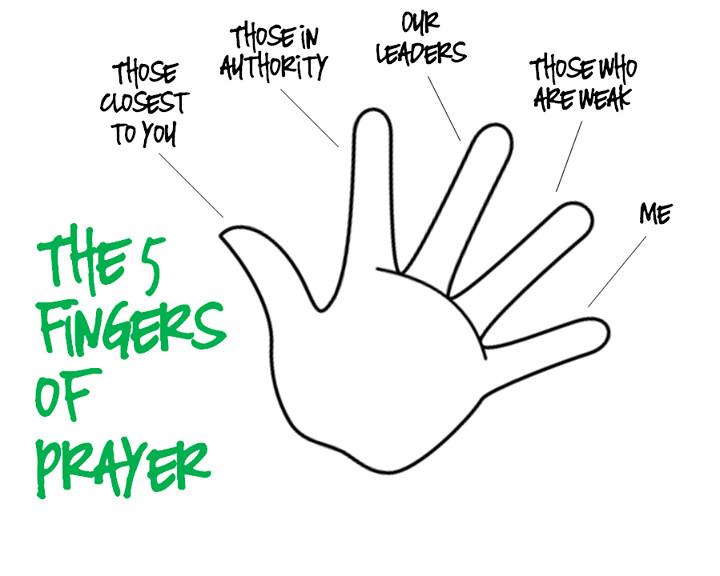The image is a simplistic, line-drawn illustration of a left hand, presented on a white background. The hand is shown palm-up, displaying a cartoon-like quality with no intricate details or textures. "The Five Fingers of Prayer" is prominently captioned in green handwritten script on the bottom left. Each finger of the hand is labeled with black directional lines leading to corresponding texts: the thumb - "those closest to you", the pointer finger - "those in authority", the middle finger - "our leaders", the ring finger - "those who are weak", and the pinky finger - "me". The central message of the image is a religious guide, indicating different groups to pray for with each finger.